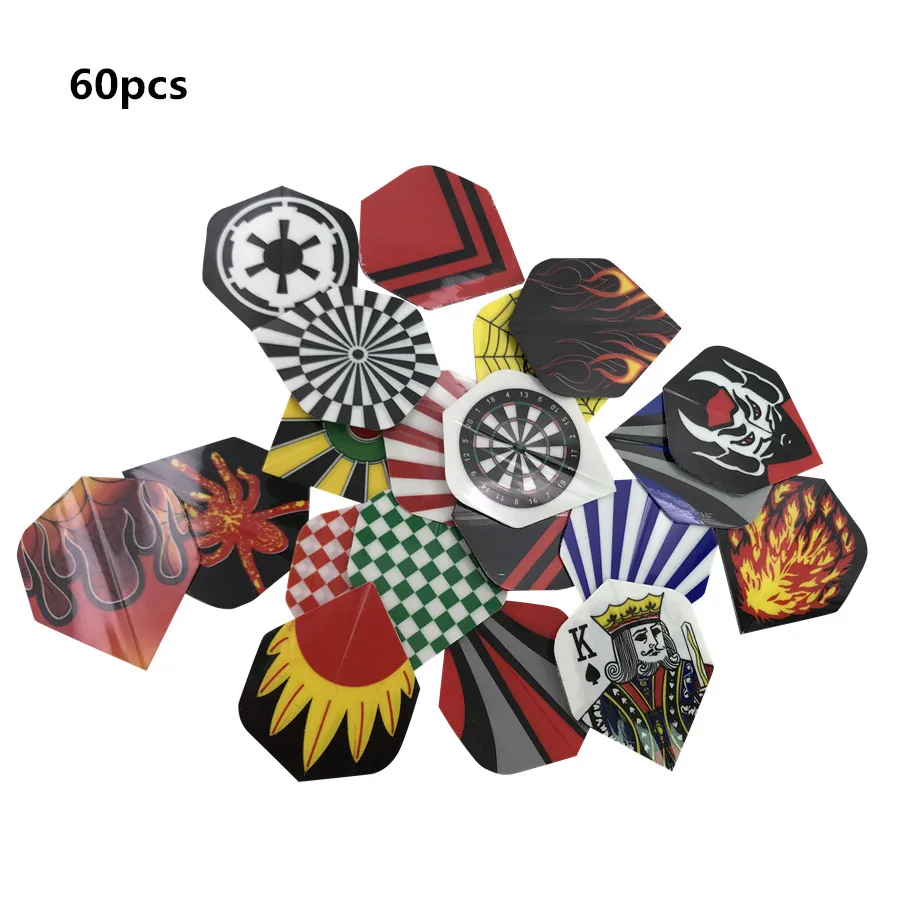A collection of 60 uniquely designed guitar picks is displayed against a white background. The picks, shaped similarly to guitar picks but with a more pointed bottom resembling a pinched hexagon, feature a variety of intricate and vibrant designs. In the upper left-hand corner, "60 PCS" is prominently displayed in black text, indicating the quantity. The illustrated patterns on the picks include a nautical steering wheel, a dartboard, the King of Spades, and both red and yellow spiders. Additionally, there are designs such as black and white radiating stripes, red and white and green and white checkered patterns, flames, a sunshine motif, black and white stars, yellow and black stripes, and more abstract designs. This detailed assortment suggests a colorful and eclectic variety suited for collectors or musicians.